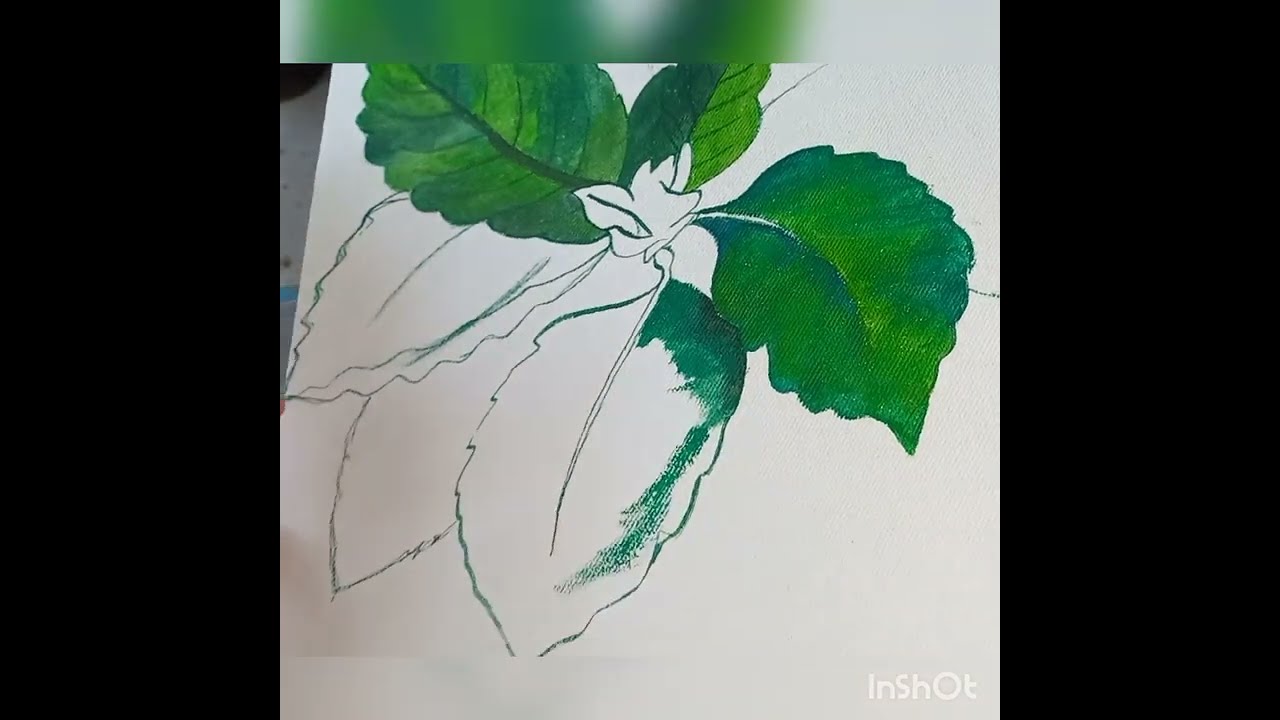The image depicts a partially completed hand-painted flower on thick, grainy white paper. The flower is fairly large and showcases six leaves, of which three and a half have been painted in various shades of green, including dark and mid-green hues. The remaining leaves are meticulously outlined, hinting at the final composition. In the center, the flower itself is outlined but remains uncolored, leaving its final hue a mystery. The background is kept clean, free of any additional elements, focusing solely on the flower. Notably, there are two black rectangular strips running vertically along the left and right sides of the paper, and in the bottom right corner, the text "NSHOT" appears in a white font, with the letters I, S, and O capitalized.